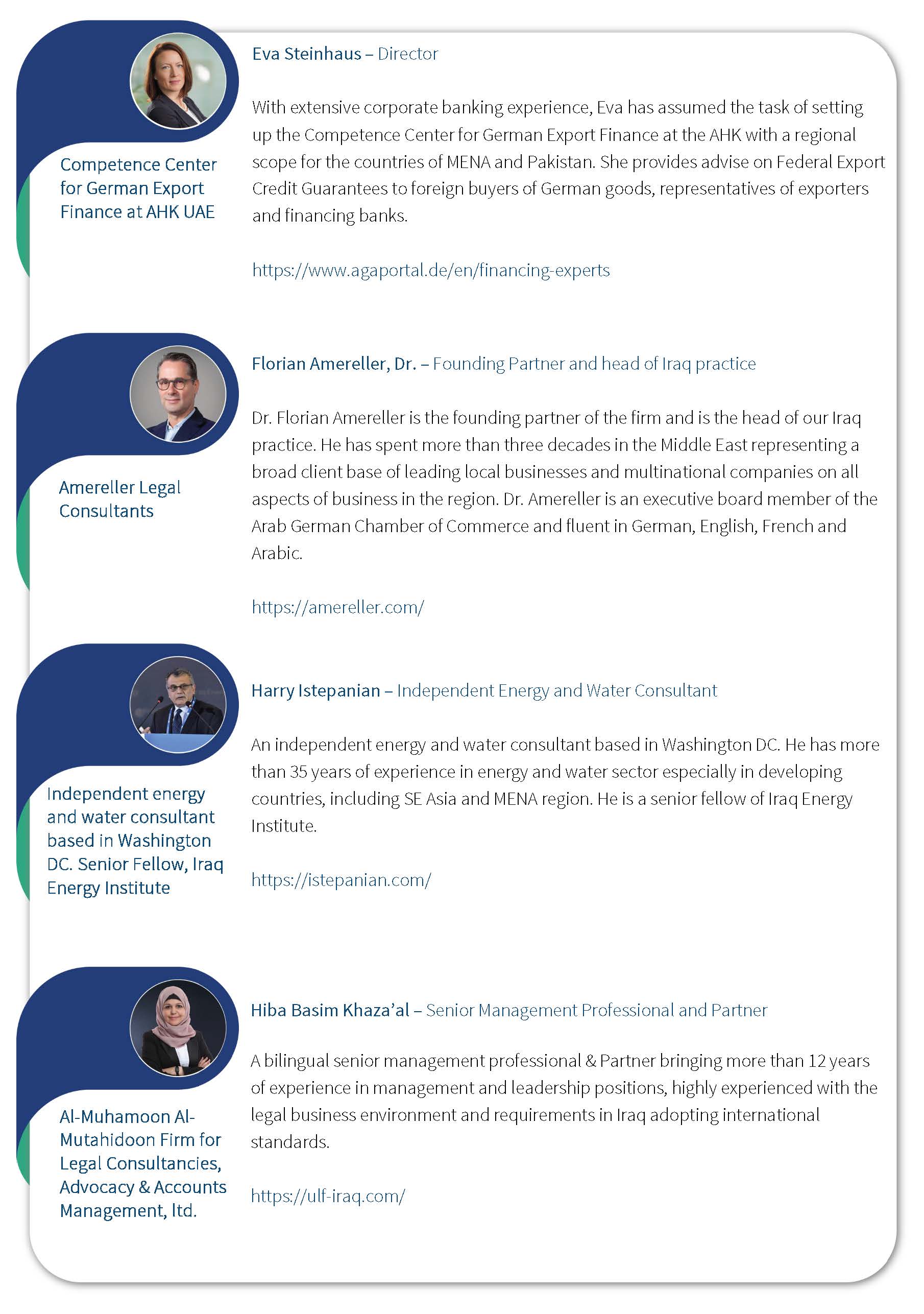Caption: 

The screenshot depicts a webpage showing the management staff, presented in a visually engaging format that resembles a resume layout. The design features four circular images aligned vertically, each representing a different team member. To the left, a graphical element curves behind a styled piece of paper with a drop shadow, giving a three-dimensional effect with rounded corners.

At the top is Eva Steinhaus, the Director of Competence Center for German Export Finance at AHK UAE. Her information is highlighted in green text under her name, accompanied by detailed black-and-white text elaborating her background.

Next is Florian Emlerler, a man wearing glasses. He holds the position of Doctor and is a Founding Partner and Head of Iraq Practice at Lemeler Legal Consultant. Below him is Harry Estepinian, an Independent Energy and Water Consultant based in Washington DC, who is also a Senior Fellow at the Iraq Energy Institute.

At the bottom is Hiba Basim-Kazal, who is described as a Senior Management Professional and Partner at Al-Muhammad Al-Mutahidum, a firm specializing in legal consultancies, advocacy, and accounts management limited. Notably, while all team members are Caucasian, Hiba Basim-Kazal appears to be of Middle Eastern descent. The webpage offers a comprehensive insight into the expertise and backgrounds of these professionals.